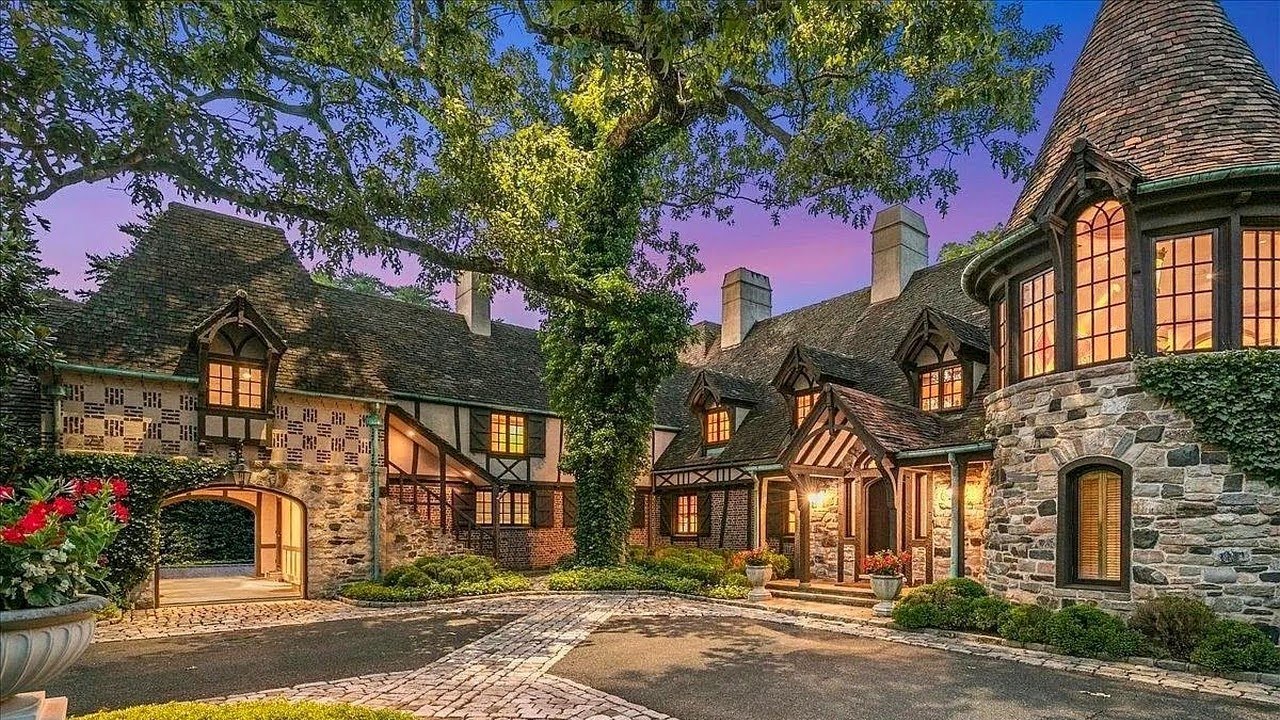This image captures a highly detailed and impeccably lit scene of a picturesque European-style mansion that exudes the charm of a French chateau. The house, which could either be computer-generated or an exceptionally photographed shot, stands with an almost surreal quality despite its hyper-realistic features. The mansion's exterior walls are predominantly constructed of multicolored gray and black stone, accented with a grayish stucco and brown support wood, adding to its rustic yet elegant aesthetic.

The structure includes a rounded turret with a sharp steeple roof and large arched windows on the right side, evoking a castle-like feel. The turret's stonework is meticulously detailed, enhancing the overall grandeur of the home. Towards the left, there is a spacious area with a prominent wooden awning over a large entrance, possibly indicating the main entryway. 

Extending further to the left is another wing of the mansion that features an arched entryway, which might serve as a drive-through or carport, given its open, tunnel-like bottom. Adding to the charm, the mansion has three steep, chimney-clad roofs that accentuate its stately appearance.

The driveway is an artistic blend of dark asphalt and stone pavers, leading up to the house and seamlessly integrating with the cobblestone area. In the foreground, a potted flower plant with red petals adds a touch of color, complementing the large tree enveloped in lush green vines that stands in front of the mansion. The entire scene is bathed in the warm hues of a sunset, with a sky that transitions from blue to pink to orange, painting a serene backdrop.

Overall, the well-balanced composition, vibrant lighting, and intricate architectural details of this mansion create a scene reminiscent of a Thomas Kinkade painting, making it a likely depiction of a luxurious hotel or a bed-and-breakfast nestled in a tranquil setting.